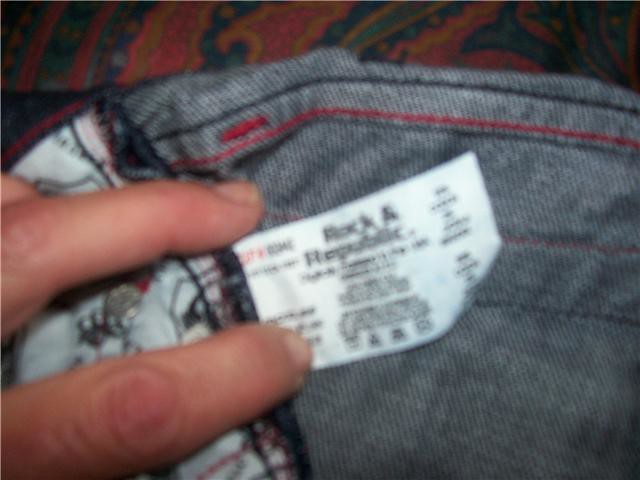The image showcases a close-up of a white clothing tag on a pair of jeans, held down for clarity by two fingers from a left hand. The denim appears to be either grey or very light blue, with visible seams along the edge of the pants. The fingers, which could use a nail trim, display knuckles that are slightly pink and perhaps mildly bruised. The jeans rest on an ornate rug with a rich red, blue, and yellow pattern, bordered by intricate designs forming a circular motif. Within the top right corner of the rug's pattern, a shape resembling a dolphin fin is discernible. Unfortunately, the text on the tag remains illegible in the photograph.